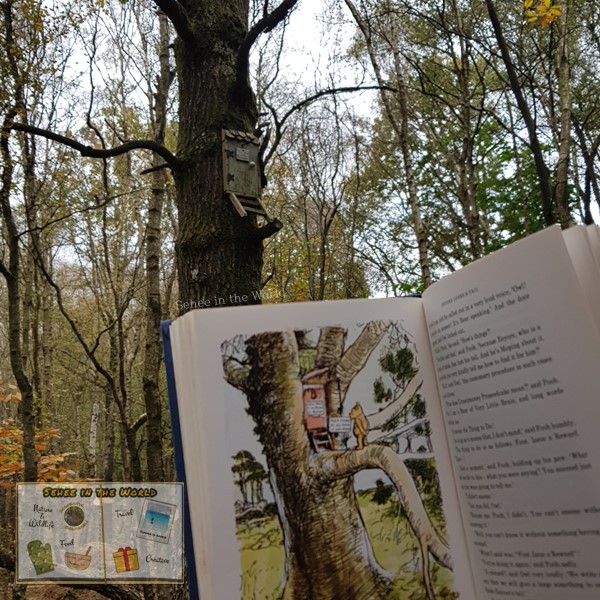The image captures a serene scene set in a wooded forest, where the foliage is transitioning into the vibrant hues of autumn. The trees are adorned with a spectrum of colors, from bright oranges and yellows to a more muted, faded green. Nestled among these trees is a wooden bird's nesting box, complete with small steps or perches leading up to it. 

In the bottom left corner, a sign is visible displaying the text "SEE HE" alongside various clip art illustrations, including a green oven mitt, a pink mixing bowl, a yellow gift package adorned with a red ribbon, and a Polaroid photograph. The focal point of the image, however, is an open book displayed against the forest backdrop. The text on the book is too blurred to read, but the left page features an illustration of a yellow bear climbing a tree towards a nesting box, mirroring the scene in the photograph. The yellow bear suggests that the book may be a story from Winnie the Pooh.